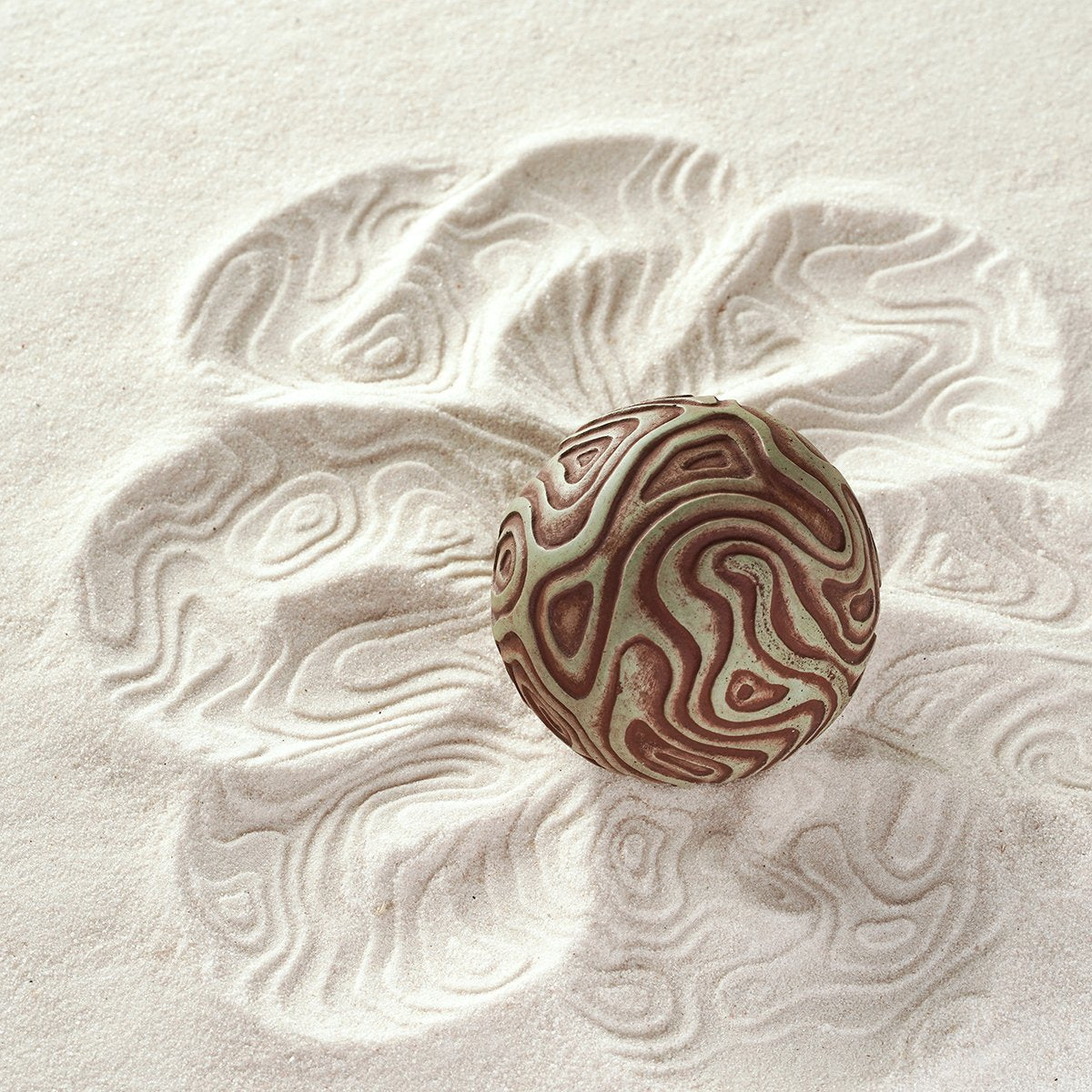The image features a cream-colored sphere with red and brown swirls and intricate carvings, approximately the size of a tennis ball. The sphere is set on a bed of sand, and it appears to have been rolled from a central spot in various directions. This movement has created multiple depressions in the sand, forming an impression that resembles a flower with the ball positioned at its center. The intricately carved designs on the sphere have transferred onto the sand, leaving a striking, sculpted pattern. The sphere is noted for its detailed and creative appearance, and its interactive nature suggests a thoughtful artistic process.